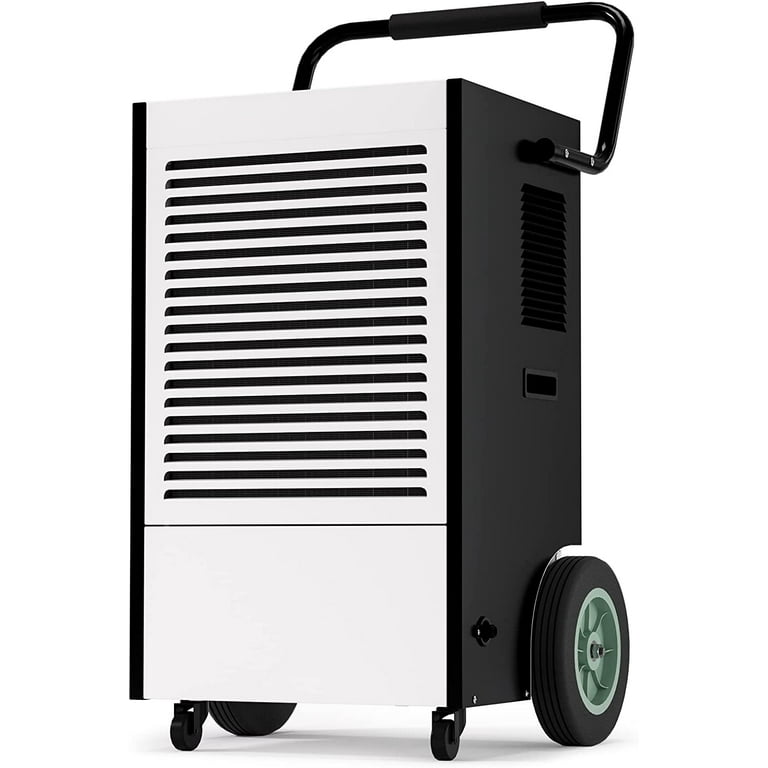The image is a photograph taken in a photo studio, showcasing a rectangular, upright mechanical device that appears to have a white front panel with black horizontal cooling vents. The front panel is divided into two white sections, with the top section featuring black vent slits and the lower section marked by a black line. The sides of the device are black, each featuring additional horizontal vents. The device is designed for mobility, equipped with two smaller swiveling front wheels and two larger rear wheels with green rims and rubber tires attached to an axle. Additionally, there is a black handle with a foam grip, allowing the device to be easily pushed or wheeled to different locations. The aesthetic and functional elements suggest a piece of equipment that could be moved conveniently, likely similar in size to luggage.